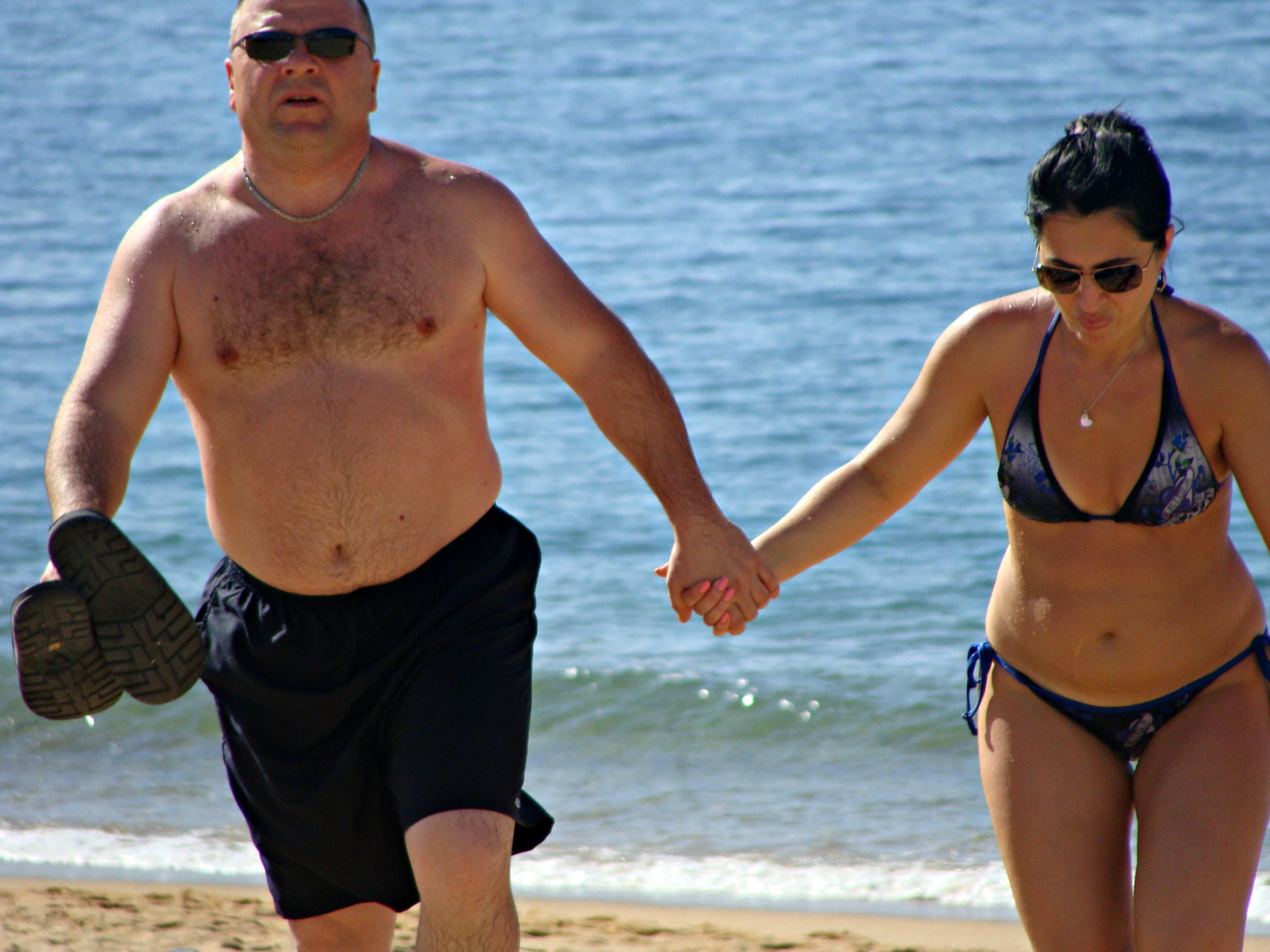The image captures a middle-aged couple, possibly in their 30s, emerging from the blue waters onto the sandy beach, walking towards the camera. On the left side is Michael Chiklis, a well-known actor and director. He is Caucasian, slightly overweight at around 250 pounds, and has a buzzed haircut hinting at balding. Chiklis sports dark sunglasses, blue-colored swimming trunks, and a tight chain necklace around his neck. He's carrying his sandals in his right hand and holding the hand of a woman with his left. The woman on the right is also somewhat overweight, around 200 pounds, with dark sunglasses and dark hair done up in a ponytail. She wears a vibrant blue bikini adorned with floral designs and accessorizes with a necklace featuring a large gem. Her nails are painted pink. The scenic background highlights the waves and water, with the beach's sand visible at the lower part of the image, emphasizing their recent emergence from the ocean.